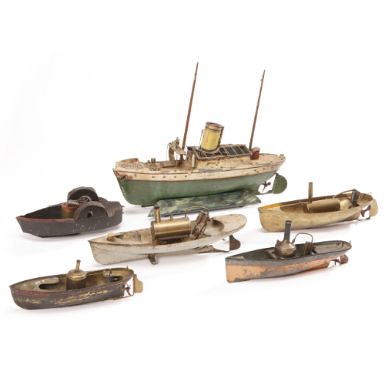The image displays a collection of six miniature sailboats, each unique and showcased against a white background. Positioned in three rows of two, the toy boats appear aged and weathered, suggesting they are models of historical ships. 

The foremost boat is black with a compact design and a distinctive small back. Behind it is the largest model, reminiscent of a cruise ship or a steamship, characterized by its light-green base, white upper structure, two prominent masts, and a raised spot between the masts that resembles a small cabin. 

In the middle row, two boats stand out: one is entirely white, featuring a prominent steel engine with a large stack resembling a barrel on the left side, while the other boat, placed slightly behind and higher, exhibits a wooden appearance with a smaller barrel-like stack at its center. 

The back row includes short, stubby grayish boat with two big round half circles on top of it, alongside another boat that is brown on the sides, gray on the top, and has a unique bong-shaped stack in the middle. 

These detailed and diverse models capture the essence of various types of boats, showcasing intricate designs and features typical of different eras.